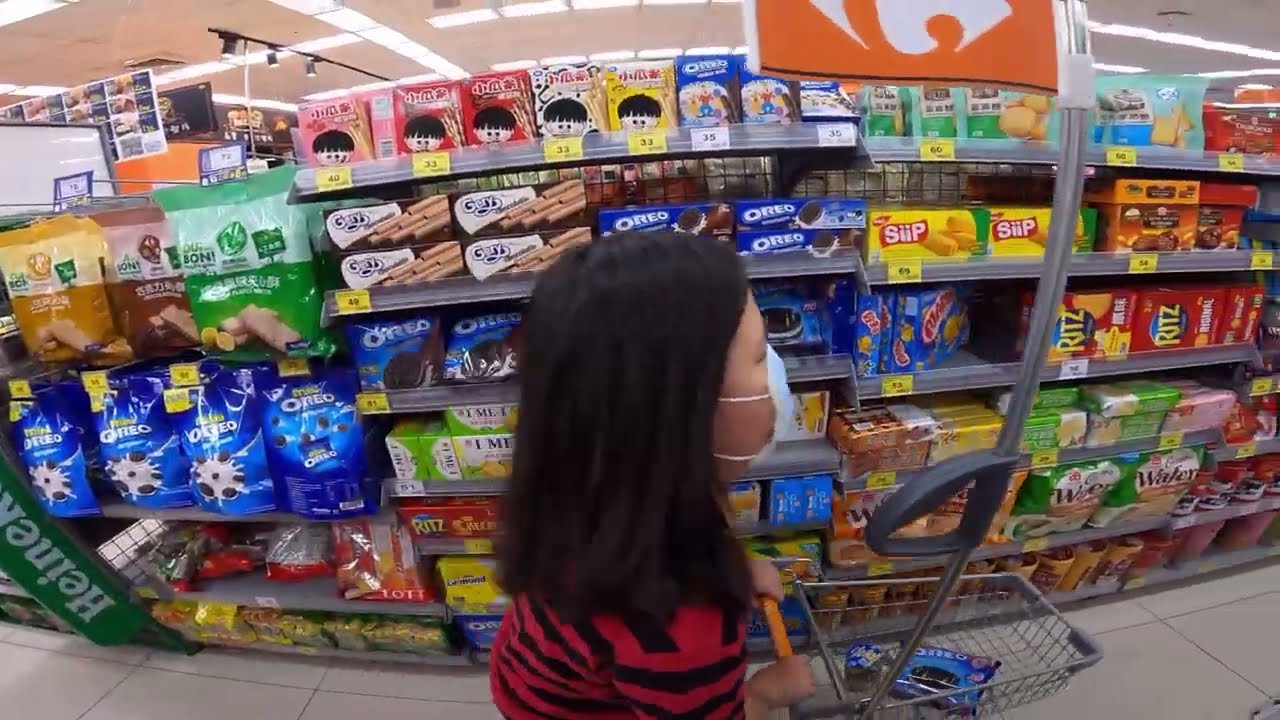In this wide rectangular photograph taken from above, an Asian woman stands in the cookie aisle of a grocery store, facing to the right. She is wearing a light blue face mask, a red and black striped shirt, and has short black hair. To her right, she pushes a small gray cart with an orange handle, which holds a bag of Oreos. A tall gray pole topped with an orange and white flag is positioned at the top right corner of the image. Behind her, a shelf displays a variety of cookies and snacks, with packs of Oreos and Ritz crackers prominently visible. A Heineken sign is spotted on the left side, adding a contrast to the otherwise snack-filled aisle.